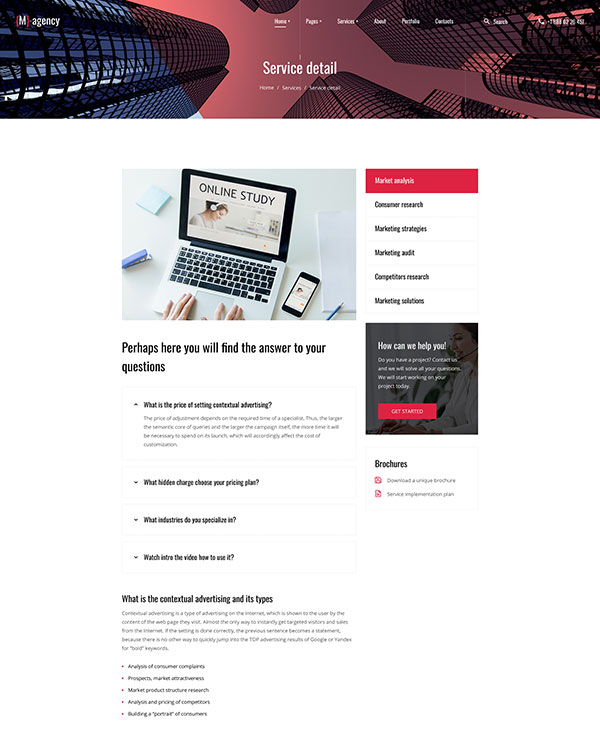### Website Screenshot Description

The screenshot captures a detailed view of a website's landing page with a modern, visually engaging design.

**Header Section:**
- **Logo:** The top header features a logo with a red parenthesis-enclosed white capital 'M', adjacent to the lowercase word "agency" in white, all aligned on a single line.
- **Background Image:** The background of the header area displays a conceptual graphic of skyscrapers viewed from below, with repeating and duplicated building shapes indicative of a stylized cityscape.
- **Overlay Design:** The left quarter of the header (approximately 25%) is tinted blue, while the remaining portion features a red overlay, both of which only mask shapes while still allowing the buildings' reflections to be visible.
- **Title and Navigation:** Centered in the middle of this header is the page title "Service Detail" in white text, accompanied by small, unclear text beneath it. The top left of the header showcases the site’s navigation menu in white text, with items including "Home," "Pages," "Services" (each with dropdown options), "About," "Portfolio," and "Contact." To the right, there's a magnifying glass icon followed by the word "Search," a telephone icon, and an unreadable phone number.

**Main Content Area:**
- **Layout:** The page adopts a two-column layout, with the left column taking up 70% of the width and the right column 30%. This main content is centered within 50% of the total page width.
- **Image and Text:** At the top of the main column, there is an image of a person using a laptop and a phone beside it, both screens displaying "Online Study" in black text on a white background. The image also includes a female-presenting figure wearing headphones and various desk items (a pencil, stapler, stack of paper, and sticky notes).
- **Informational Text:** Beneath the image, a phrase reads, "Perhaps here you will find the answer to your questions," followed by four collapsible dropdown sections containing bolded questions and answers in smaller, plain text.
- **Additional Content:** Further down, a section titled "What is contextual advertising and its types" begins an illegible text portion due to resolution, accompanied by five small red bullet points.

**Secondary Column:**
- **Links and Resources:** The narrower column on the right includes several links: 
  - "Market Analysis" in white text on a red background at the top.
  - Five more links in black text on white backgrounds, likely including topics like "Consumer Research," "Marketing Strategies," "Marketing [something]," "Competitors Research," and "Marketing Solutions."
- **Support Section:** A black box containing the header "How can we help you?" in larger, bold white text and an accompanying red button (possibly labeled "Get Started") with further smaller, unreadable text.
- **Brochures:** Below this, another box labeled "Brochures" with two small red icons and corresponding text in black, all too small to be discernible.

The page is structured to guide the user through various informational sections efficiently, with a blend of bold visuals and functional navigation, despite the difficulty in reading certain details due to image resolution limitations.